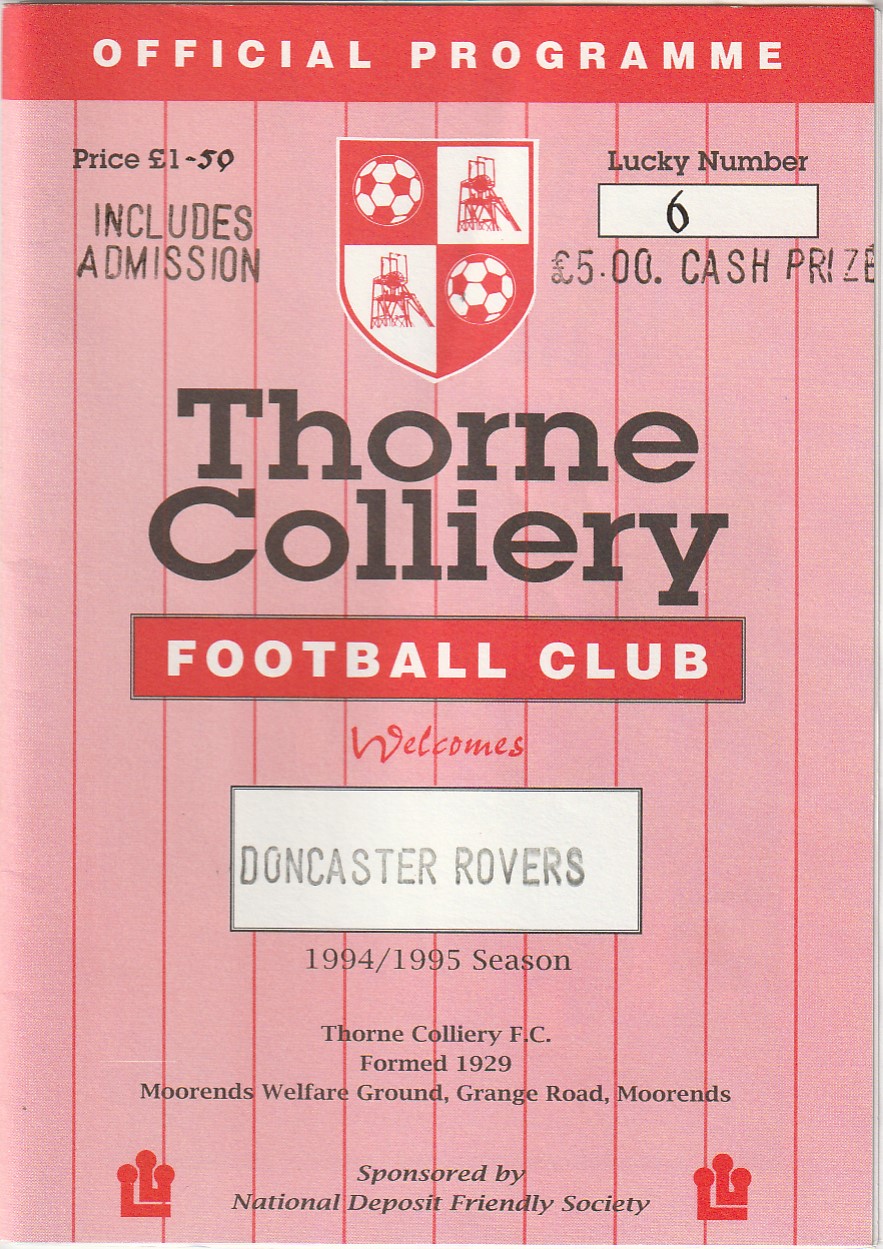This image depicts the front cover of a vintage program booklet for the Thorn Colliery Football Club from the early to mid-90s. The cover features a light red, almost pink hue, adorned with vertical red stripes, giving it a distinctive striped pattern. At the very top, a red box contains white text that reads "Official Program". Below this, there is a four-part crest featuring two soccer balls and two chairs. The cover announces: "Thorn Colliery Football Club welcomes Doncaster Rovers for the 1994-1995 season". Additional text reveals that the club was formed in 1929 and is based at the Moran's Welfare Ground on Grange Road, Moran's. Sponsored by the National Deposit Friendly Society, the program also mentions the price of $1.50, which includes admission, and notes a lucky number 6 offering a $5 cash prize. The colors present in the image include shades of pink, red, white, black, and gray. The booklet occupies the entirety of the image, emphasizing its significance as an official document for the soccer team.